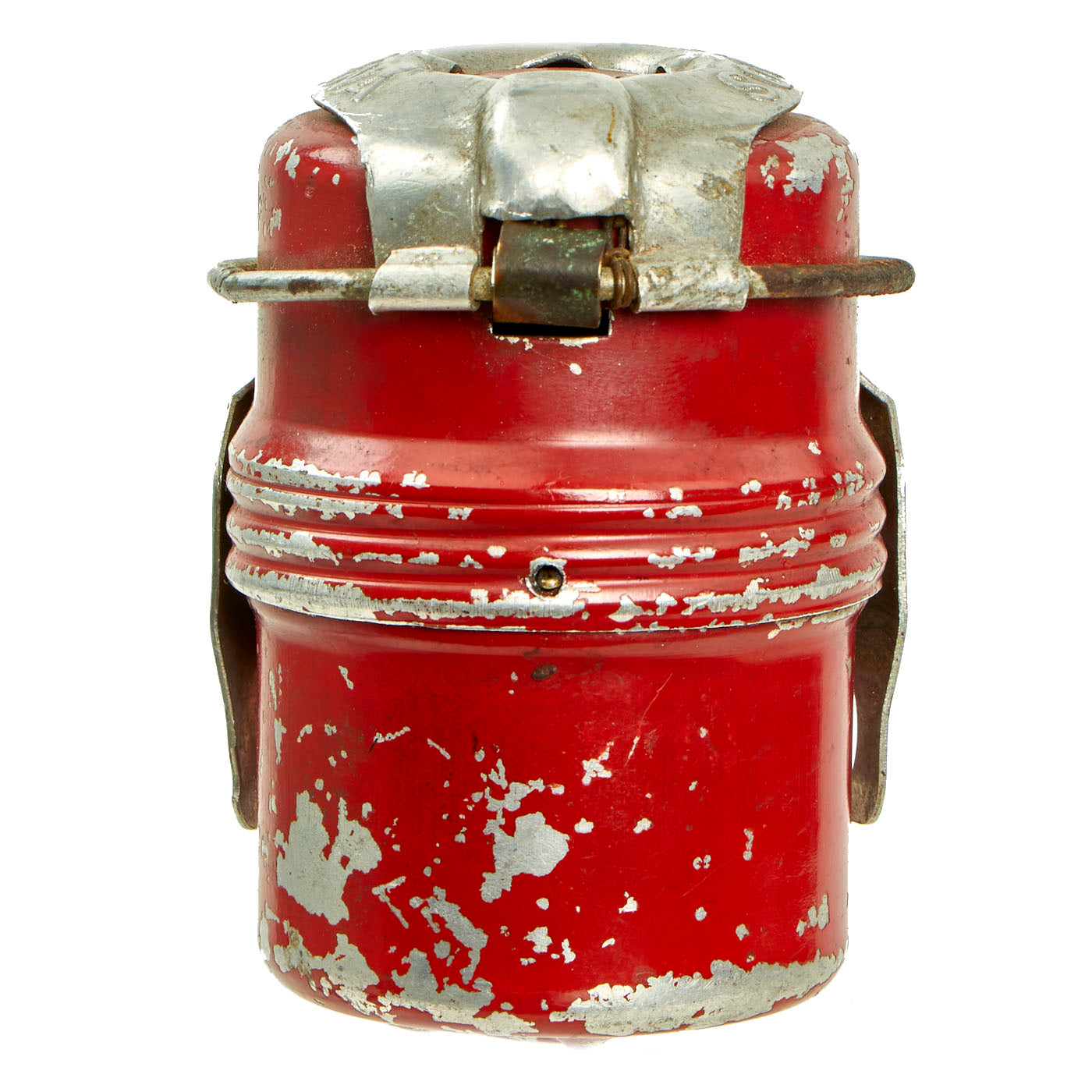This image displays an antique red canteen with significant paint chipping revealing a silver-colored, likely aluminum or steel, base material. The canteen features a twist-off lid of the same metallic hue, with noticeable rust and wear. Characteristic of its old age, both the body and the lid display extensive rusting and peeling paint, indicating it hasn't withstood the test of time well. The canteen has a distinctive structure with three horizontal ridges around its center, where the most paint wear has occurred. It also includes two metallic handles on either side, with evident rust on the wire hinges. In the center of the canteen lid, there is a tiny golden-colored hole. All these features are set against a stark white background, emphasizing the aged and worn condition of the object.